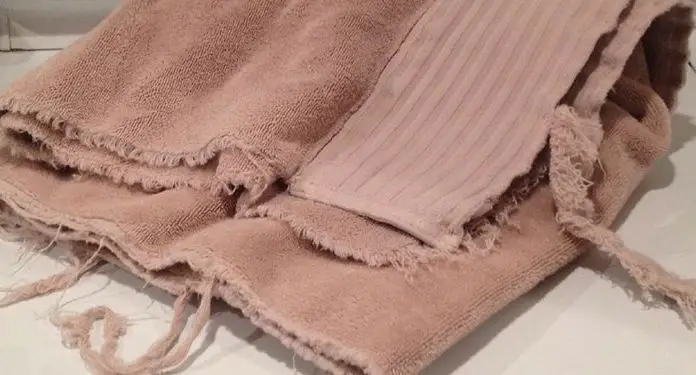The image depicts a close-up of a light salmon or peachy pink-colored towel, evidently old and worn. The towel is placed on a flat, white surface, which could be a floor or table, casting shadows beneath and to the right, suggesting the presence of overhead lighting. The towel’s edges are heavily frayed and shredded, with visible wool and yarn strands falling out, indicating significant wear and age. Despite its tattered state, the towel appears clean and has been folded twice, revealing a distinction between the main soft part and a smoother, non-terry cloth trim along one edge. The fabric’s worn and torn sections further reinforce the towel's long-term use and abandonment.